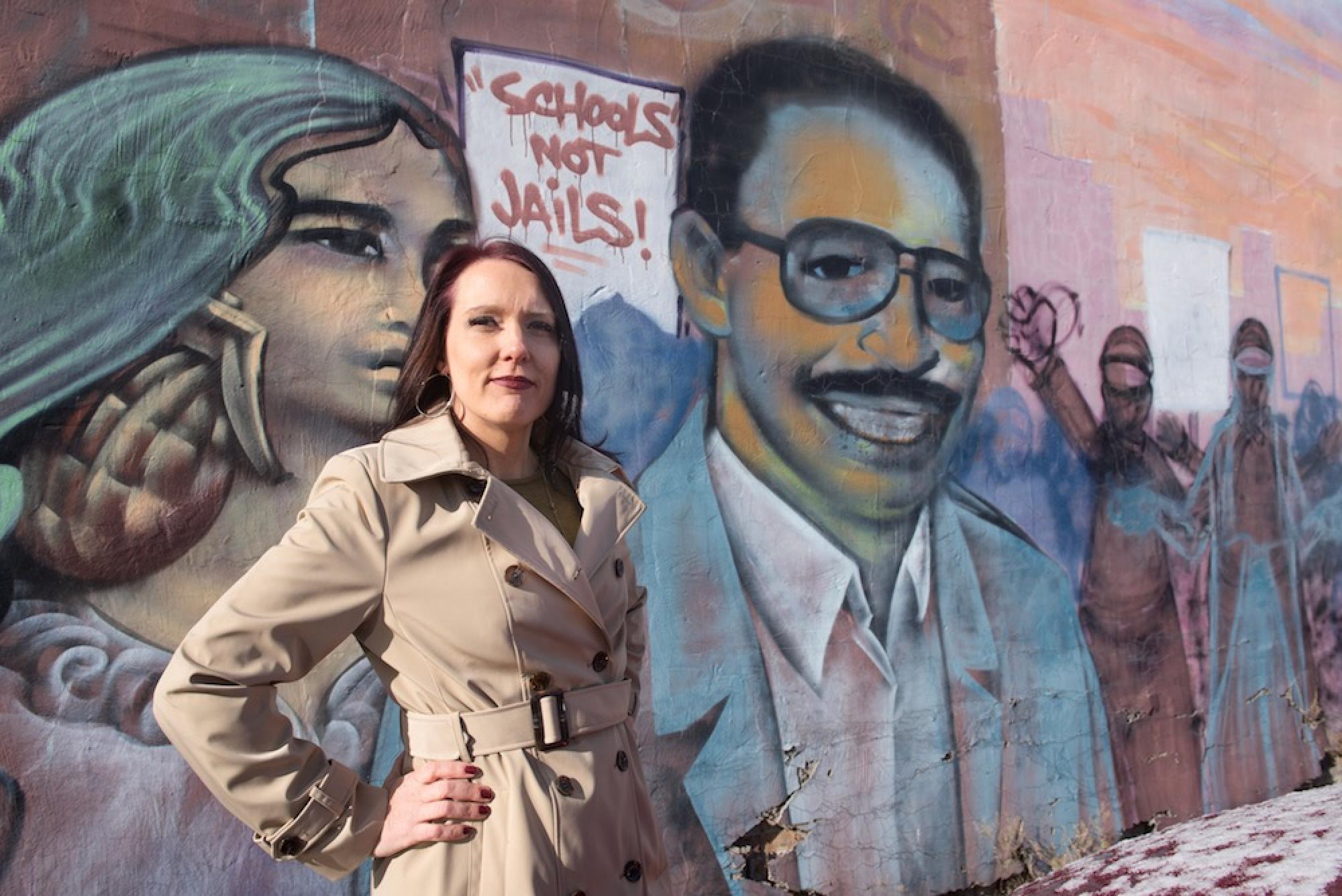In the image, a white woman with black hair stands confidently in front of a vibrant, politically charged mural, dressed in a light tan trench coat with her left hand on her hip. The mural, painted on a city wall, spans multiple thematic sections. On the left side, it features two prominent African-American figures: a woman declaring "Schools Not Jails" in red text with underlines and a smiling black man, both symbols of the need for better educational resources. Meanwhile, the right side showcases two men with pink visors, one fist-pumping and the other walking in a blue, translucent robe amidst a devastated cityscape, possibly representing resistance and struggle. The mural's colorful and complex imagery, set against an orange and purple sky, echoes a strong political message about the militarization and inequity in the U.S. school system, framing the woman standing before it as a possible participant in a broader protest or social commentary.